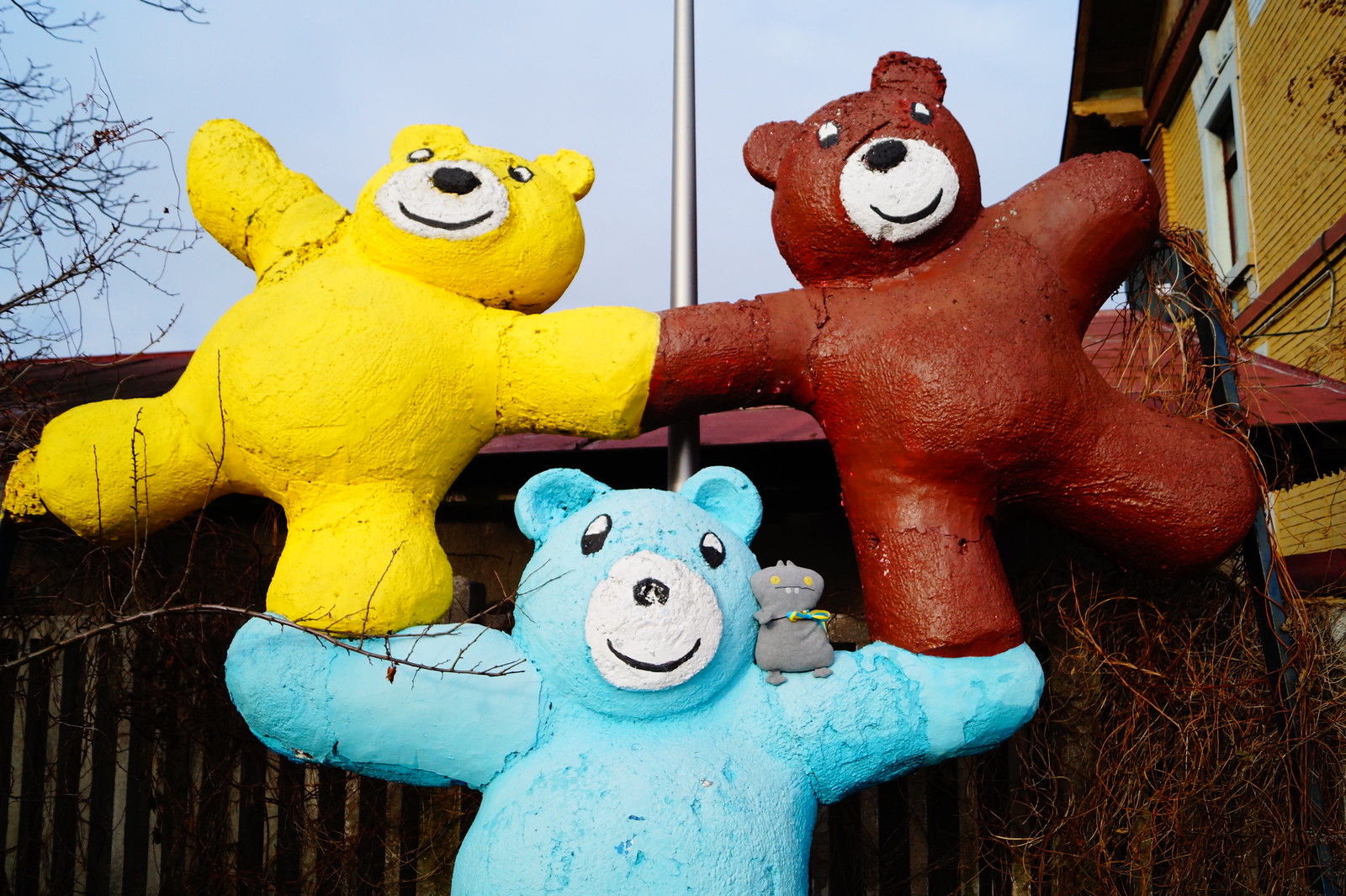The image depicts a whimsical outdoor scene centered around three teddy bear statues arranged in a playful formation. In the foreground stands a light blue teddy bear with outstretched arms, featuring white around its mouth and a black nose, mouth, and eyes. This blue bear supports two smaller bears on its arms: a yellow bear with a white face and black nose on the left, and a brown bear with a white snout, black nose, and eyes on the right. Both smaller bears extend their paws toward each other as if holding hands. Perched on the blue bear's right shoulder is a small grey creature with orange-yellow eyes and a lime-green bow tie, adding a whimsical touch.

The background reveals a bluish-grey sky, punctuated by a metal pole that rises vertically through the center of the frame. On the left side, scraggly tree branches are visible, while on the right side stands a yellow, two-story clapboard house with a new paint job. A wooden fence with nearby scraggly bushes runs horizontally across the image's backdrop, completing the charming outdoor scene.